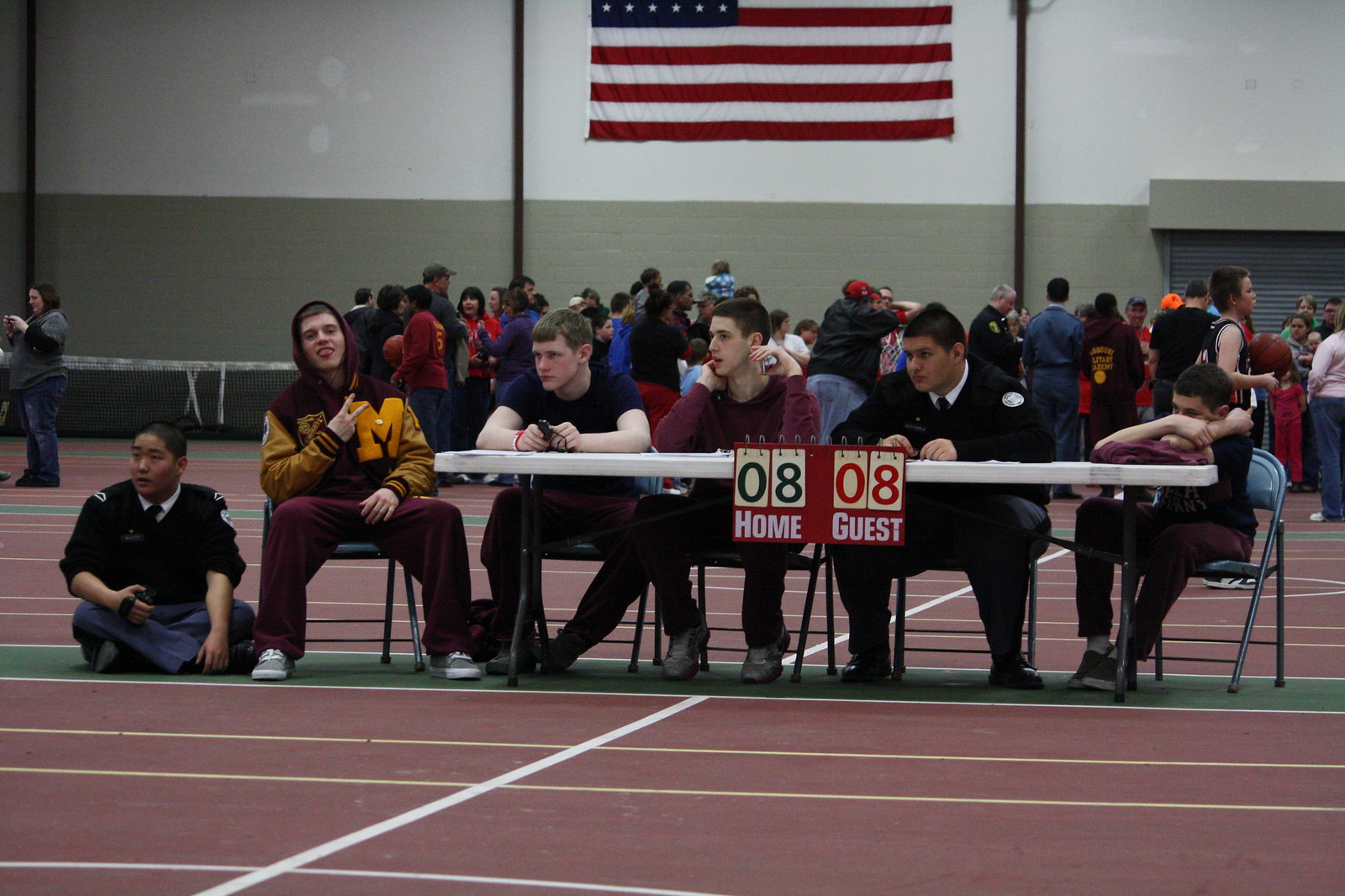In this full-color indoor photograph taken at a sports event, we see a distinctive scene dominated by a scorekeeper's table with six young men, around 17 or 18 years old, positioned around it. The floor beneath them is reddish, resembling a track. A strip of green with a table on it runs along the area, and a red banner hangs from the table displaying the numbers 08 Home and 08 Guest, indicating a tied score.

Behind the table sits a group of five young men on chairs, while one man sits cross-legged on the floor in front, dressed in a uniform with gray pants, a black top, and a shaved head. This uniformed individual appears to be part of an ROTC team and is holding an object in one hand. 

On the table, there are four visible scorecards, and the individuals behind it are engaged in their roles. On the far left, a boy in a dark-colored T-shirt keenly watches the ongoing activity. Next to him, another youth in a maroon sweatshirt is perched attentively. The actual scorekeeper sits centrally, dressed in a dark suit with a dark tie, his short brown hair neatly trimmed. On the far right, a boy in a varsity jacket with a bright yellow 'M' and maroon-colored sweatpants has his hood up, and he is making a V sign for victory.

The backdrop features a gray wall that transitions into white halfway up, adorned with the bottom half of an American flag and surrounded by a crowd of spectators, adding to the atmosphere of this engaging sporting event.